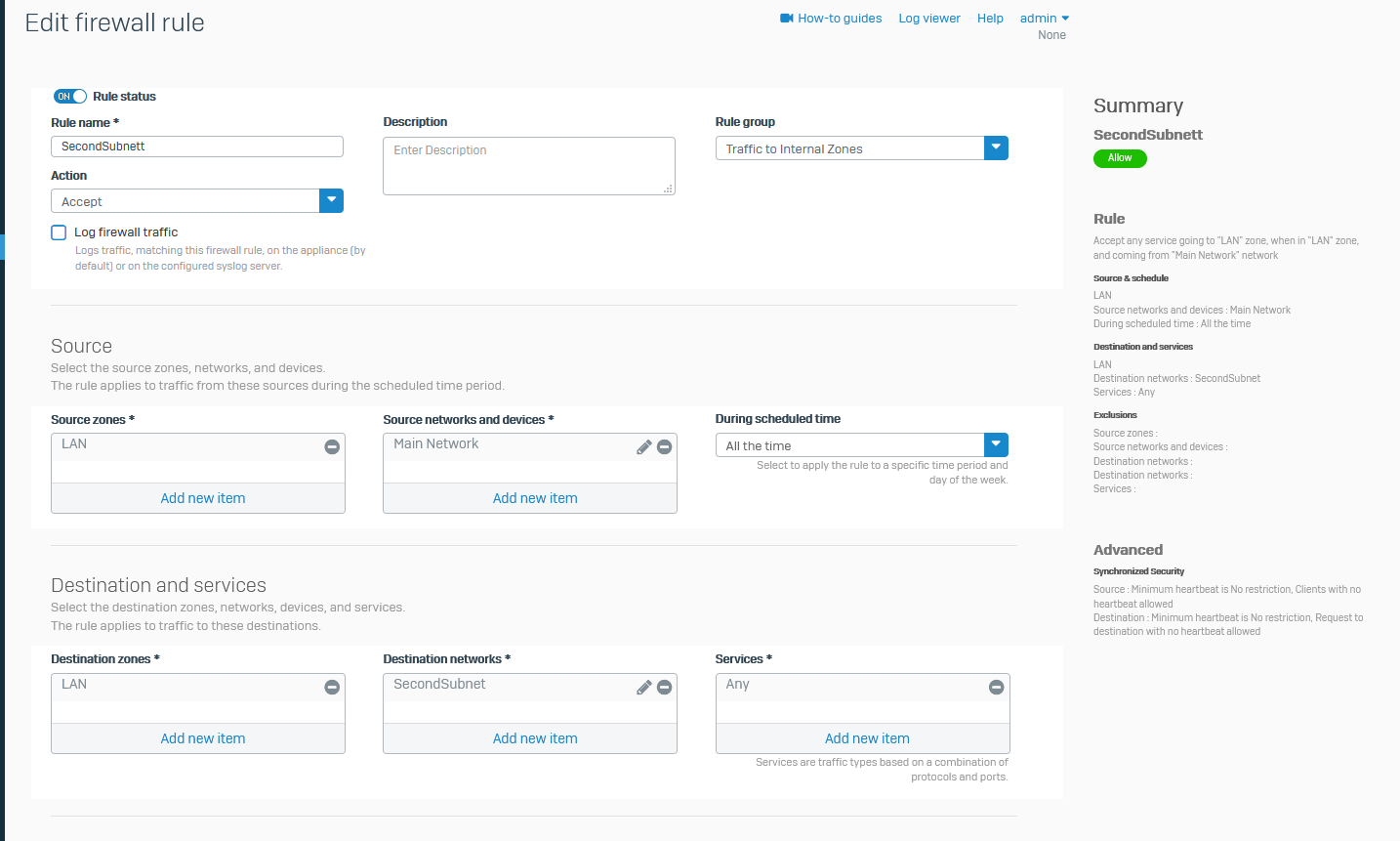Screenshot of a Firewall Rule Editing Interface

This screenshot captures a web interface for editing a firewall rule on an unknown website. The header contains navigation options including "Edit Firewall Rule" on the left and "How-to Guides," "Log Viewer," "Help," and "Admin" on the top right.

The main section of the interface is dedicated to configuring the firewall rule. Key elements include:

- **Rule Status**: The rule is currently turned "On."
- **Rule Name**: "Second Subnet."
- **Subnet Description**: Option to enter a description for the subnet.
- **Rule Group**: "Traffic to Internal Zones."
- **Action**: Set to "Accept."
- **Log Firewall Traffic**: Logs traffic matching this firewall rule by default on the appliance or the configured syslog server.

**Sources**:
- **Source Zones**: "LAN," with an option to "Add New Item."
- **Source Networks and Devices**: "Main Network," with an option to "Add New Item."
- This rule applies to traffic from these sources during the specified time period.

**Scheduling**:
- The rule is set to apply "all the time," but there is an option to select a specific time period and day of the week.

**Destinations and Services**:
- **Destination Zones**: "LAN," with an option to "Add New Item."
- **Destination Networks**: "Second Subnet," with an option to "Add New Item."
- **Services**: "Any," with an option to "Add New Item." Services are defined based on a combination of protocols and ports.

**Summary Panel** on the right:
- Displays a concise summary of the rule:
  - **Rule Name**: "Second Subnet" (spelled as S-E-C-O-N-D S-U-B-N-E-T-T).
  - **Action**: "Allow."
  - **Source**: "LAN Zone," "Main Network," active "all the time."
  - **Destination**: "LAN Zone," "Second Subnet."
  - **Services**: "Any."
  - **Exclusions**: Various exclusions for source zones, source networks and devices, and destination networks.
  - **Advanced Synchronized Security**:
    - **Source**: Minimum heartbeat restriction not set; clients with no heartbeat are allowed.
    - **Destination**: Minimum heartbeat restriction not set; destinations with no heartbeat are allowed.

This detailed overview of the firewall rule editing interface provides insights into the specific configurations and options available for managing network traffic.